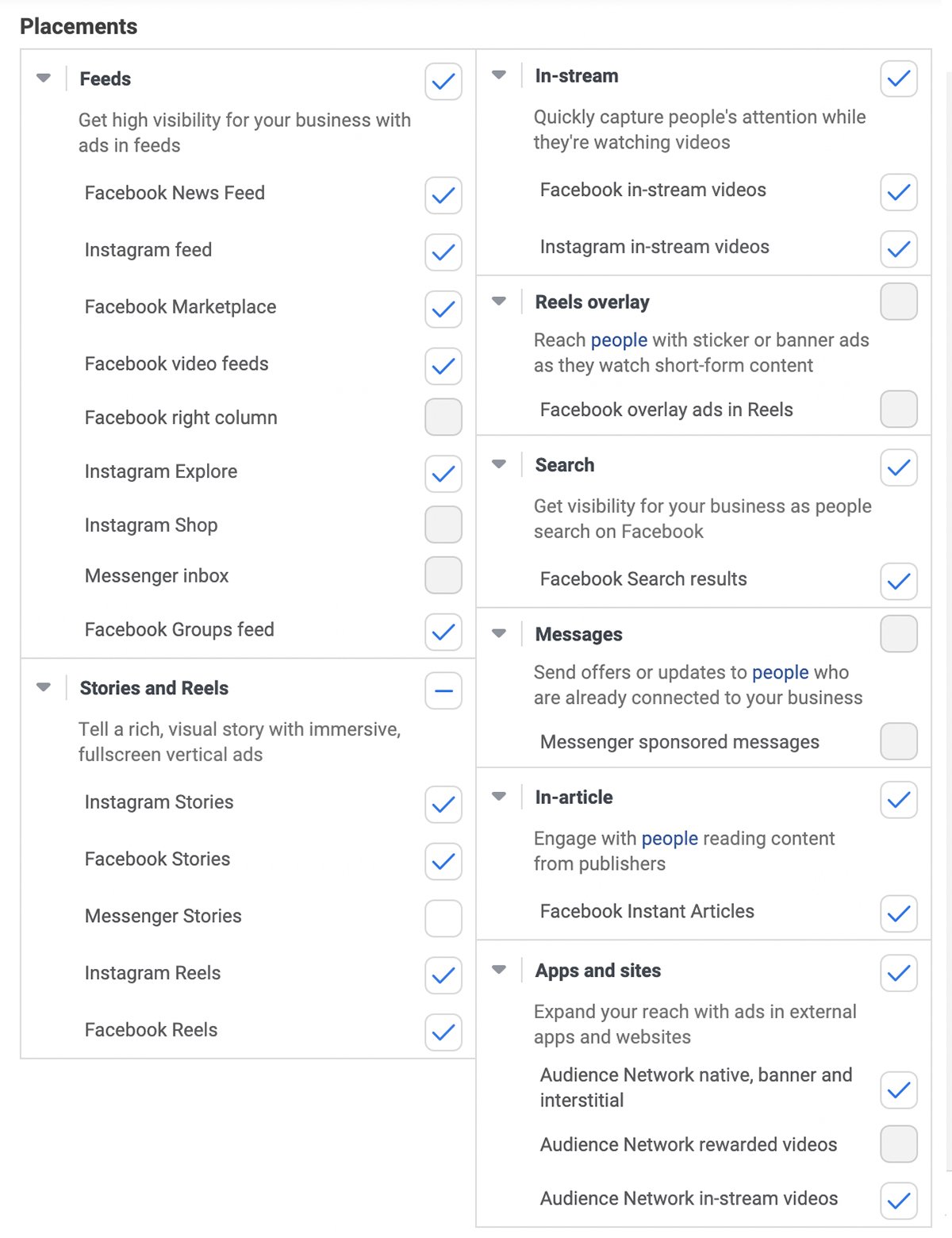This image captures a screen displaying a detailed ad placement interface, organized into columns and rows. 

At the top, there's a section labeled "Placements" with checkboxes on the right for selecting ad locations, accompanied by explanatory text on the left. The layout features two primary columns divided into different categories. 

The first category, "Feeds," is highlighted by the statement "Get high visibility for your business with ads in feeds." A blue check mark indicates selections under this category. The Facebook News Feed, Instagram Feed, Facebook Marketplace, and Facebook Video Feeds are all checked. In contrast, the Facebook Right Column isn't selected, marked by an empty gray square. Instagram Explore is checked, while Instagram Shop and Messenger Inbox lack check marks.

As you scroll down, there's a section titled "Stories and Reels," accompanied by the description "Tell a rich visual story with immersive full-screen vertical ads." Although there isn't a checkbox section associated with this description, individual placements are detailed below. Facebook Groups Feed has a check mark, whereas Stories and Reels categories are marked with a negative sign. Instagram Stories and Facebook Stories both have check marks, whereas Messenger Stories does not. Additionally, both Instagram Reels and Facebook Reels are selected.

On the right side of the image, there's a mirror of this setup, reiterating the placement options and their respective selections with check marks.